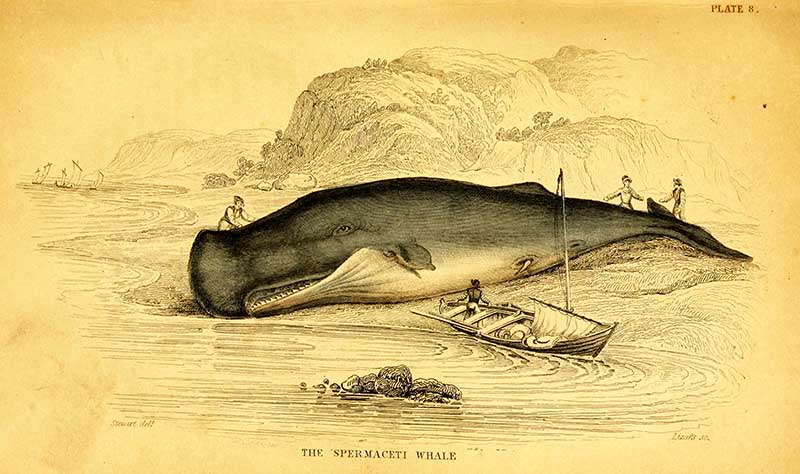This sepia-toned, monochromatic engraving depicts a massive spermaceti whale, spelled S-P-E-R-M-A-C-E-T-I, beached on a shore. The paper's yellowish tint suggests the artwork is quite old, possibly hundreds of years. Central to the image is the gargantuan whale, lying with its mouth slightly ajar, pointing towards the left. Surrounding the whale are several individuals: one near its head, two at its tail, and another in a small boat nearby, all seemingly inspecting the creature. In the background, gentle waves lap the beach, which features some grass and scattered plants. Rocky formations with a few bushes also rise behind the whale, providing a rugged coastal backdrop. Additional boats are faintly visible on the horizon. The image is titled "The Spermaceti Whale" as indicated by the text at the bottom, adding to the historical and educational nature of the illustration.